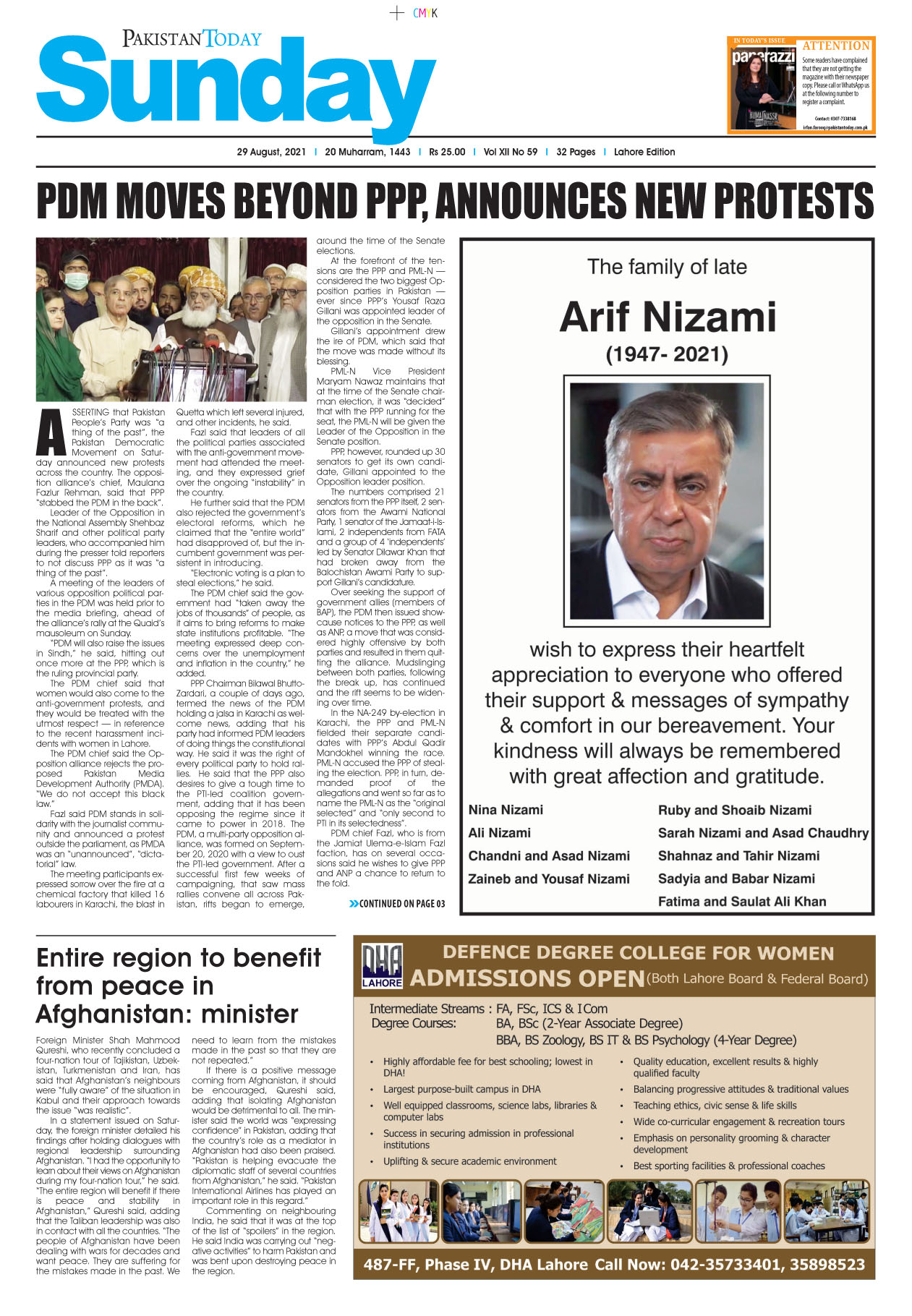**Newspaper Front Page:**

**Pakistan Today: Sunday Edition**

**Headlines in Blue:**
**PDM Moves Beyond PPP; Announces New Protest**

**Main Image:**
A photograph captures a group of men and women donned in traditional Islamic attire, gathered to deliver an impassioned speech, indicating the political climate and recent announcements from the PDM (Pakistan Democratic Movement).

**Memorial Section:**
_The Family of the Late Arif Nizami (1947 - 2021)_

A tribute section honoring the late Arif Nizami, accompanied by his photograph. The family extends their heartfelt appreciation to everyone who offered their support and messages of sympathy and comfort during their time of bereavement. The note conveys that the kindness shown will always be remembered with great affection and gratitude.

**Additional Article:**
_Entire Region to Benefit from Peace in Afghanistan, says Minister_

A report highlighting the minister's statement on the potential regional benefits that a peaceful Afghanistan could bring, emphasizing the significance of stability in the area.